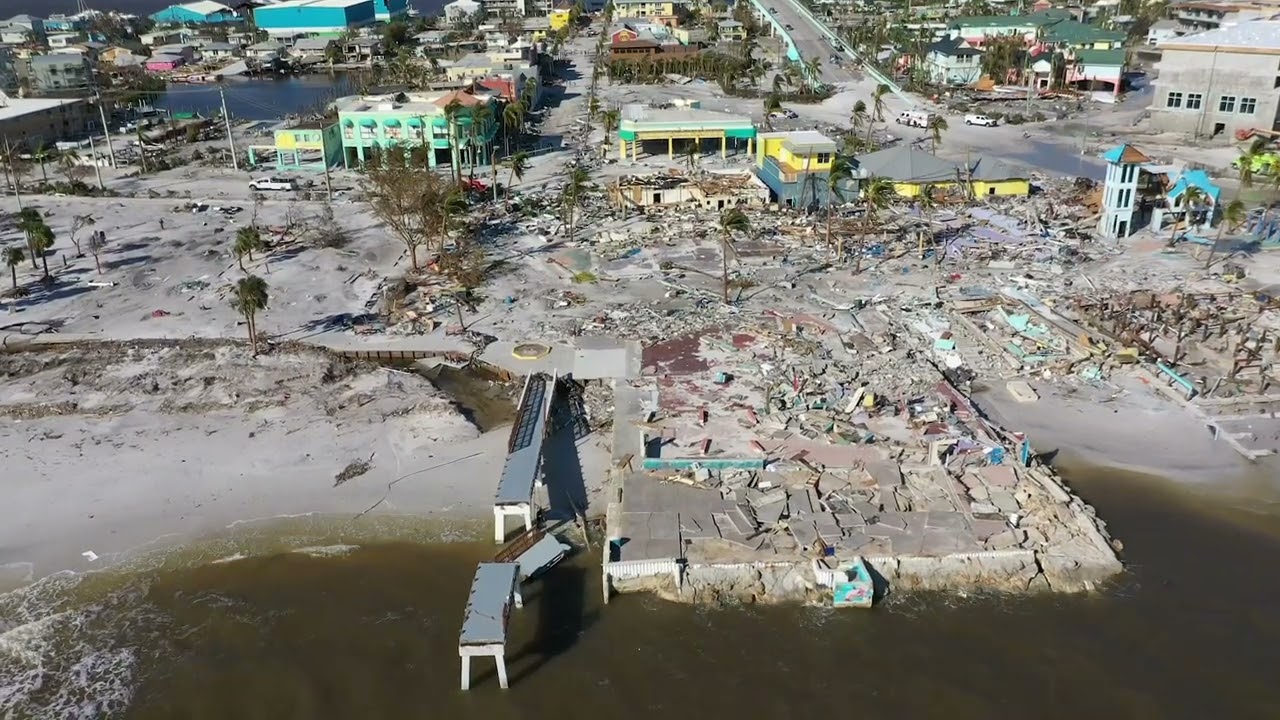This is a horizontally aligned rectangular aerial photograph capturing the aftermath of a major disaster, likely a hurricane, in what appears to be a beach town. At the bottom left corner, gentle white-tipped waves meet the shoreline, with water that looks dark and murky brown. The midsection of the image reveals a devastated landscape with broken concrete pieces scattered across the land, hinting at the severe damage inflicted. Some scattered trees stand amidst this chaos, and further into the background, there is a highway visible in the distance. Intact buildings can be seen on the left and right sides, bathed in daylight. Visible brightly-colored structures in aqua, light green, and bright yellow accent the far background, in stark contrast to the damaged buildings closer to the shore. A destroyed boardwalk is partially visible amongst the debris. In the upper left corner, a small pond or lake with grayish-blue water can be seen. The scene is devoid of people, underscoring the severity of the destruction.